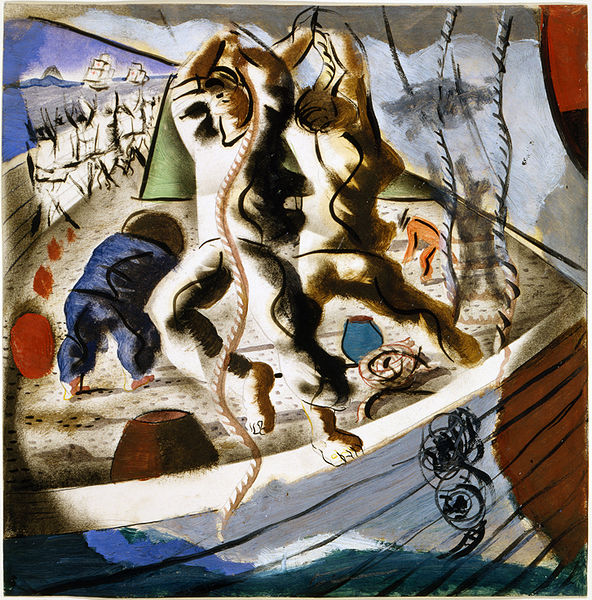This detailed, abstract, and modernistic drawing depicts a brown wooden boat featuring various shades of black, white, gray, blue, brown, orange, and peach. At the front of the boat, two men, characterized by their abstract and squiggly forms, appear to be climbing down from the mast or are engaging with a brown rope. These figures meld black, white, and brown hues in their undefined features.

Towards the back of the boat, on the left side, there's a man in a blue outfit, seemingly bent over, possibly cleaning the deck. His brown hair is faintly visible as seen from behind. To the right, another man in an orange outfit, wearing a brown and black hat, mirrors this bent-over posture, also appearing to clean the deck.

In the upper left background, additional three-masted ships float far out to sea, enhancing the nautical theme. The sail on the right upper corner of the drawing shifts from white at the bottom to gray towards the top, with ropes extending out, adding to the complex, abstract details of the artwork. The lower part of the boat, beneath the feet of the depicted characters, shows white and gray wood planks transitioning into brown, with an indistinct black swirly drawing on the lower stern. A mix of abstract shapes, including a brown vase and a blue vase or bucket along with orange circles, populates the scene, contributing to the overall abstract, modern feel of the drawing.